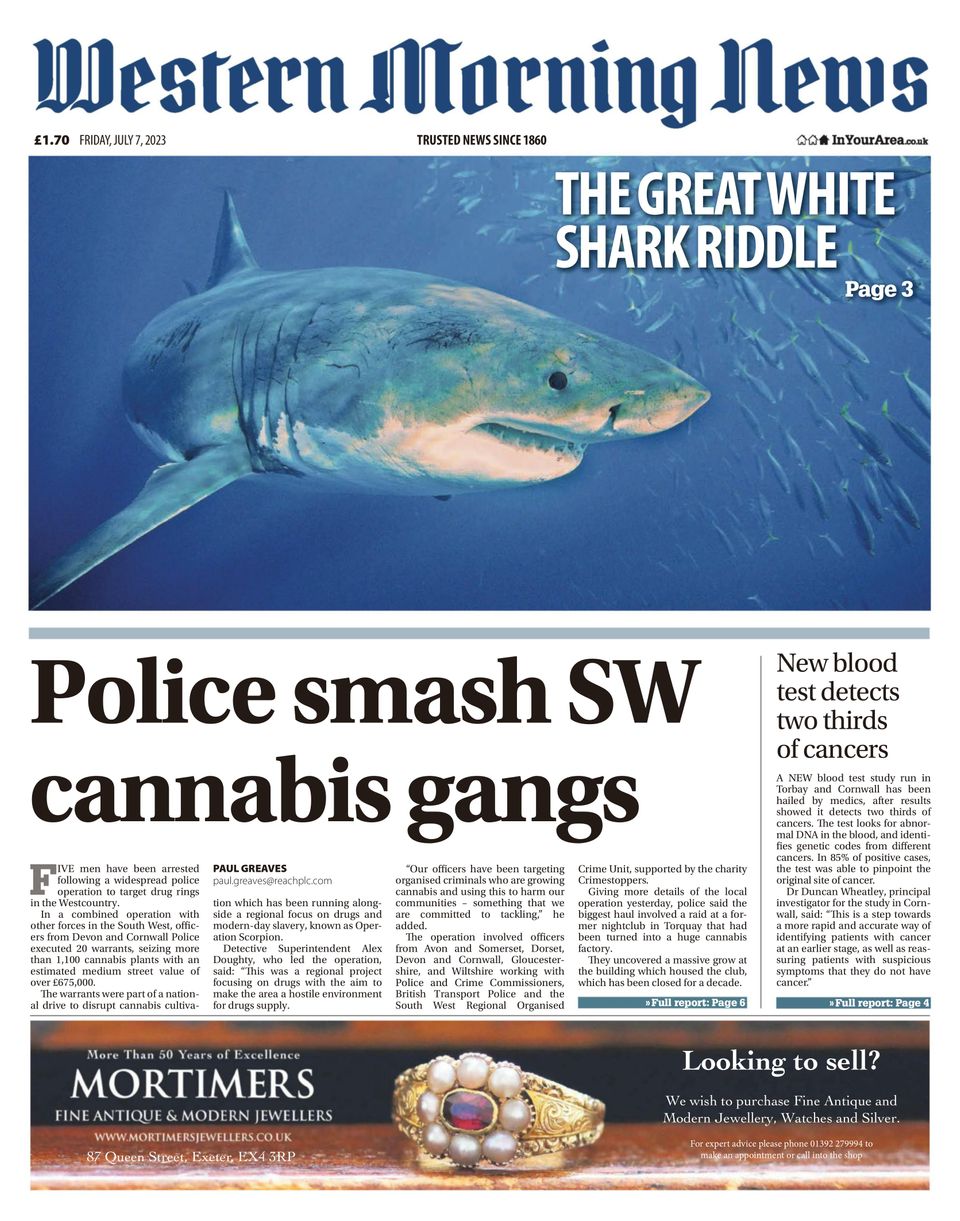The front page of the Western Morning News, dated Friday, July 7, 2023, priced at £1.70, prominently features a striking image of a great white shark swimming in blue waters amid a school of fish, accompanied by the headline "The Great White Shark Riddle" in bold white text, indicating that the full story can be found on page 3. Below this main headline, an article titled "Police Smash Southwest Cannabis Gangs," written by Paul Greaves, is visible. To the right, a smaller headline reads "New Blood Test Detects Two-Thirds of Cancers," noting that research in Torquay and Cornwall has yielded impressive results. At the bottom of the page, there is an advertisement for Mortimer's Fine Antique and Modern Jewelers in Exeter, featuring a detailed image of a lavish gold ring adorned with pearls surrounding a central ruby. The newspaper, established in 1860, proudly declares itself as trusted news in a traditional blue old English font.